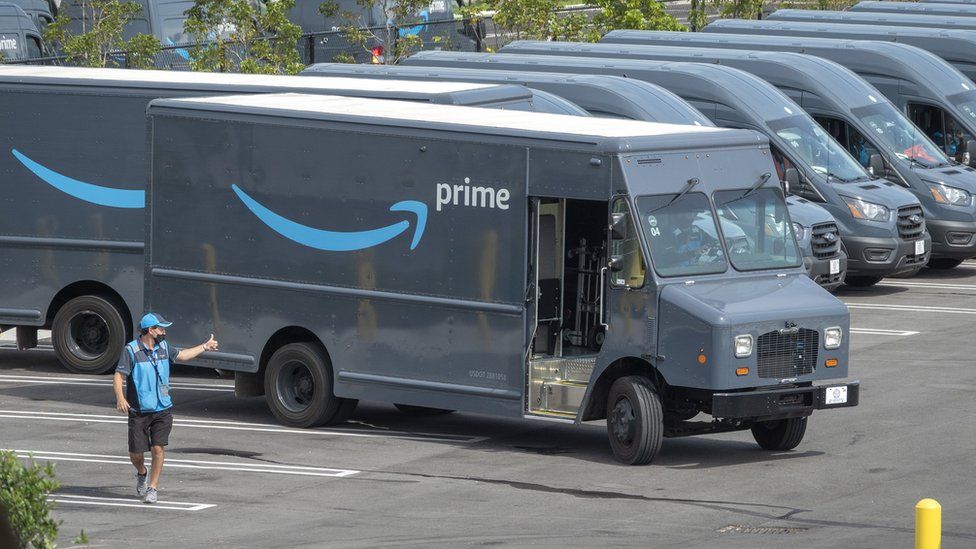In this vivid color photograph taken outdoors, the focal point is a bustling asphalt parking lot marked with white parking lines. Numerous Amazon Prime delivery vans are lined up in the lot, prominently featuring the recognizable gray vans with blue swoop curved lines and the iconic Amazon arrow. Dominating the foreground is a slightly angled Prime van, its windshield somewhat blurry with a discernible driver inside. The passenger door of this van is open, suggesting imminent departure or recent arrival. 

Next to the van, a person is captured mid-movement, walking away while glancing back and giving the driver a thumbs up with his left hand. Dressed in a blue and gray baseball cap and matching short sleeve shirt, he also wears a black face mask, a lanyard hanging around his neck, and sports dark gray shorts paired with sneakers. The scene extends beyond the vans to reveal a chain link fence adorned with green foliage, adding a touch of nature to the industrial setting. In the bottom right corner of the photograph, part of a yellow pylon is visible, adding a splash of color to the monochromatic tones of the parking area.